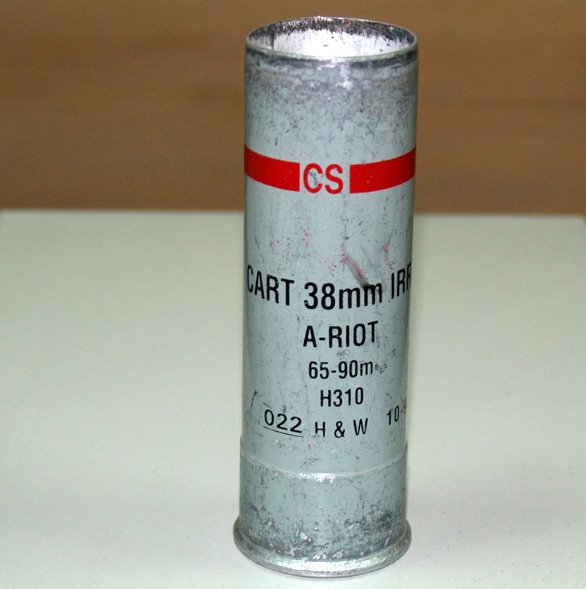The image depicts a small, narrow silver tube with dark gray speckles, hinting at the beginning stages of rust. Encircling the top part of the tube is a distinct red strip bearing the letters "CS" in red font. Below this, in black capital letters, it reads: "CART 38 mm IR," though the full word is partially obscured by the curvature of the tube. Additional markings include "ARIOT 65-90M H 310022 H & W 10." The tube is situated on a smooth, white surface, providing a stark contrast to its metallic, slightly tarnished appearance.